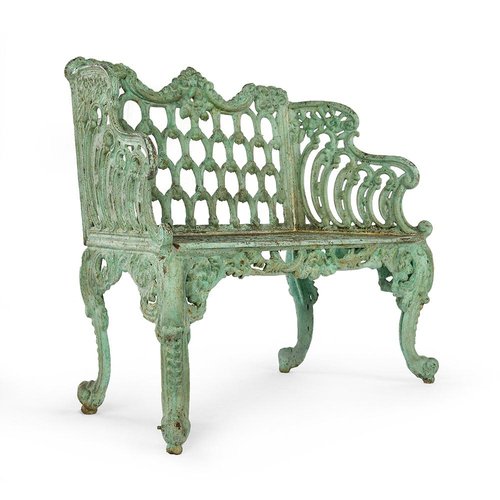The image features a very old, heavily oxidized green metal bench, likely made from copper or cast iron. This ornate bench, which could seat two people, stands out against a plain white background. Its design is reminiscent of a royal setting, with elegantly detailed and curved legs that connect via intricately decaled supports. The armrests curve gracefully upwards, meeting a backrest adorned with intricate patterns and artistic holes, giving it a woven appearance. The top of the backrest features a distinctive swoop downwards before rising into an ornate point at the center. Every element of the bench, from the handrails to the feet, showcases extensive craftsmanship and elaborate detailing, making it a striking centerpiece.